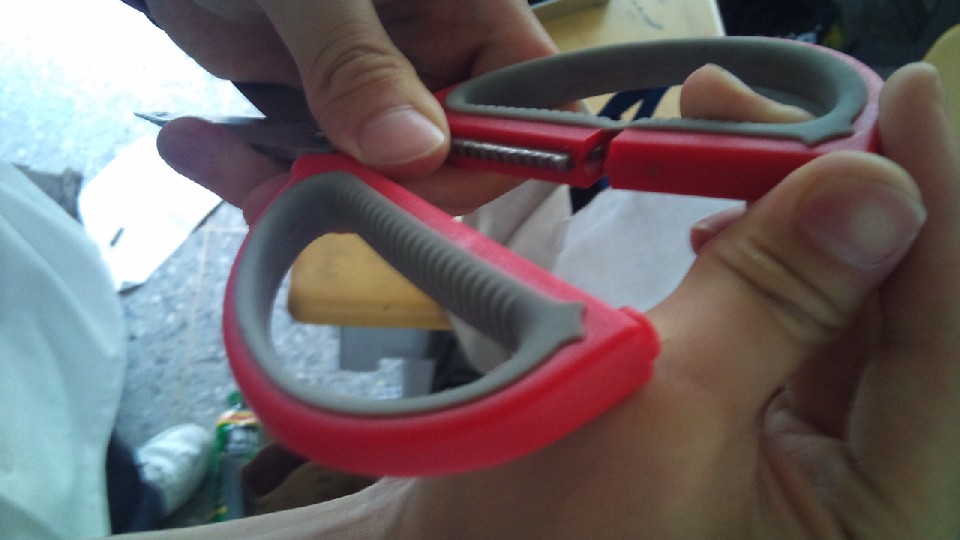This detailed close-up photograph depicts a male figure's hands holding a broken pair of scissors. The red and gray-handled scissors appear prominently in view, with one handle visibly snapped and also one handle's grip showing damage near an indent or a hole. The individual's left hand, clad in a presumably light blue or white shirt, grips the blade section directly, while the right hand is inserted in the partially broken handle, illustrating the scissors' damaged state. The setting is photographed from an overhead perspective, focusing on the hands and scissors, whilst faintly showcasing the individual’s white shoe atop a mottled gray tiled floor. The photo suggests a hands-on examination, adding a context of potential repair or demonstration of the broken tool.